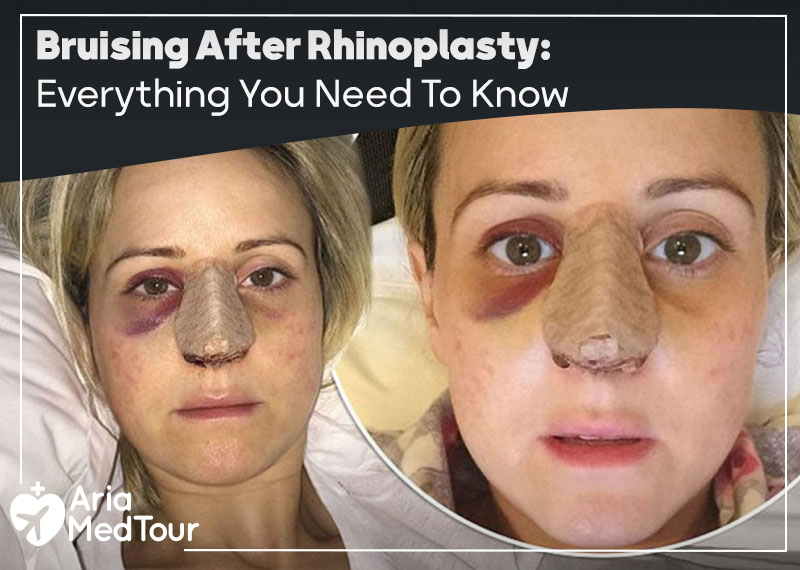The image is a poster or slide about rhinoplasty, titled "Bruising After Rhinoplasty: Everything You Need to Know" in white letters against a black banner at the top. It features two photographs of the same woman post-operation. In both pictures, she has a brown bandage covering her nose and noticeable bruising around her eyes. The left photograph, depicting her with blonde, slightly brown hair and brown eyebrows, shows her with more severe purplish bruising around her right eye and slightly less on her left. Her cheeks appear flush with a hint of rosacea. She's wearing a white top and lying on a white pillow. The right photograph, a close-up, appears to have been taken a couple of days later, showing reduced bruising that has turned more pinkish. In this image, she's wearing a plaid top. At the bottom left corner of the poster, it says "Aria Med Tour" next to a logo featuring a white heart with a cross and an airplane icon.